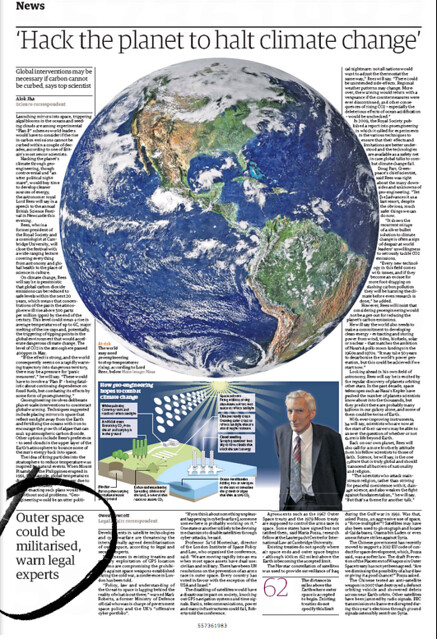This newspaper page features a prominent headline declaring “Hack the Planet to Halt Climate Change.” At the center of the page is a detailed illustration of the Earth, prominently displaying the United States and Canada. However, Canada is obscured by a blanket of clouds. Other regions visible on the globe include the Bahamas and parts of Africa, surrounded by swirling white patterns suggestive of weather systems or atmospheric interventions.

Below the globe, there is a smaller inset box containing additional text and an image. The image features an older man dressed in a dark suit, a white shirt, and a distinctive multi-colored checked tie. He stands authoritatively, likely underscoring the gravity of the accompanying text, which discusses the advent of geoengineering as a countermeasure to climate change. The passage explains a specific geoengineering method involving the burial of pipes in the ground to harness geothermal energy, which can then be used for heating homes or providing hot water.

Additionally, the article touches on the potential militarization of outer space, with legal experts weighing in on the risks and implications of such actions. The text suggests general caution, noting that the militarization of space might not be a beneficial course for humanity. The accompanying print appears quite fine and likely difficult to read without magnification.